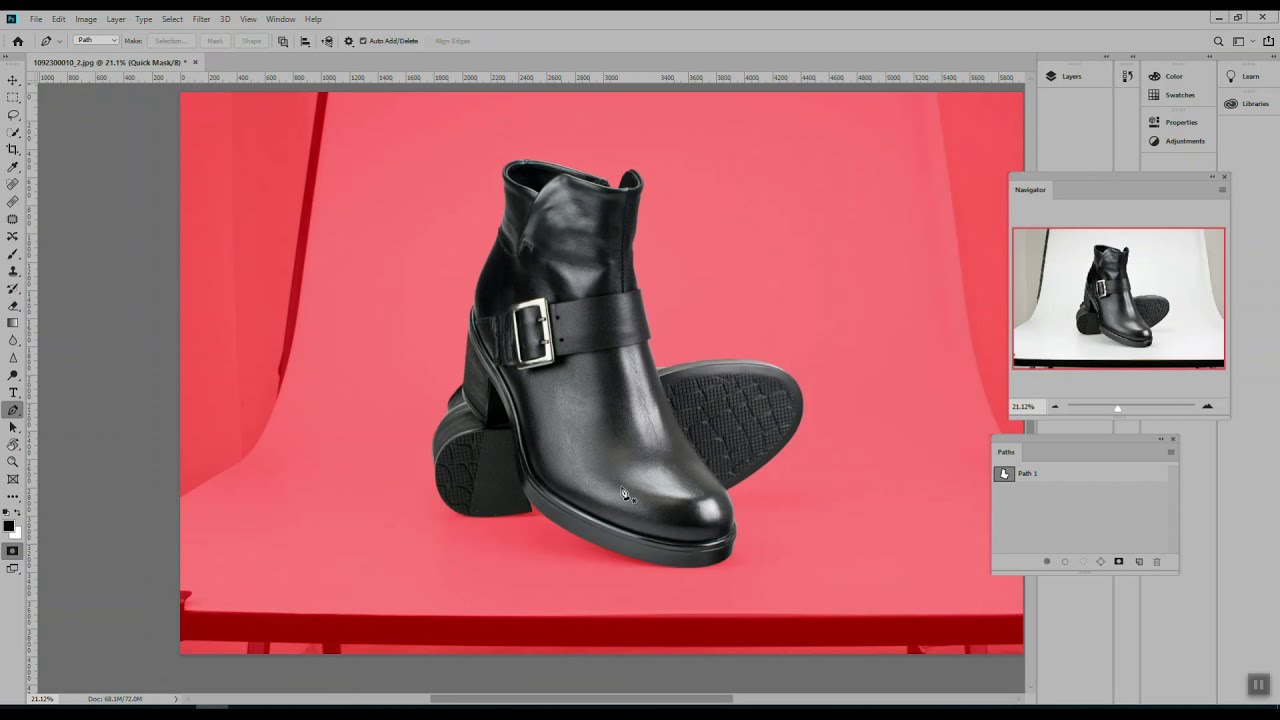This is a horizontally aligned screenshot from an image editing program, likely Photoshop or a similar application, with the typical gray interface. At the top left of the screen, the menu options "File," "Edit," "Image," "Layer," "Type," "Select," and others are clearly visible, while a vertical toolbar featuring various drawing icons runs along the left side.  

At the center of the screen is the main focus of the editing work—a photograph of women's black ankle-high boots, one positioned upright and the other laying on its side. The boots, which have silver buckles and short heels of around one to two inches, are staged on a red, slide-like background that curves downward. In the lower section of this red background, the boots are prominently displayed, suggesting they might be part of an advertisement. 

To the right of the edited image, there's a smaller panel showing the original version of the photograph on a white background, likely artist's easel paper, positioned in the same staged manner. Grayish curtains can also be faintly seen framing this smaller preview, hinting at the original setting of the photo shoot.